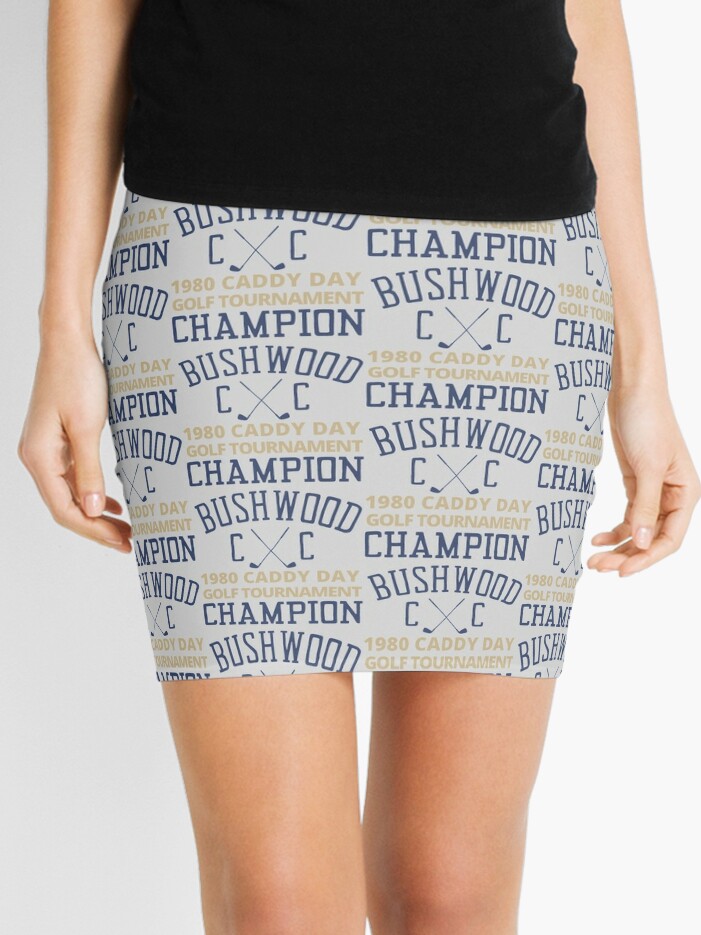In this detailed advertisement image, we see the lower half of a white woman from her abdomen down to just below her knees. She is standing against a white background, wearing a black shirt and keeping her arms naturally by her sides. The focal point is a white cotton skirt adorned with a repeating pattern. The pattern features the words "Champion Bushwood" in black or blue capital letters, followed by an "X" formed by two crossing golf clubs. To the left and right of the crossed clubs are capital letters "C." Below this, in capital letters, it says "1980 Caddy Day Golf Tournament." This design is consistently repeated across the entire skirt, creating a visually engaging and thematic garment suitable for casual outings or golf-related events.